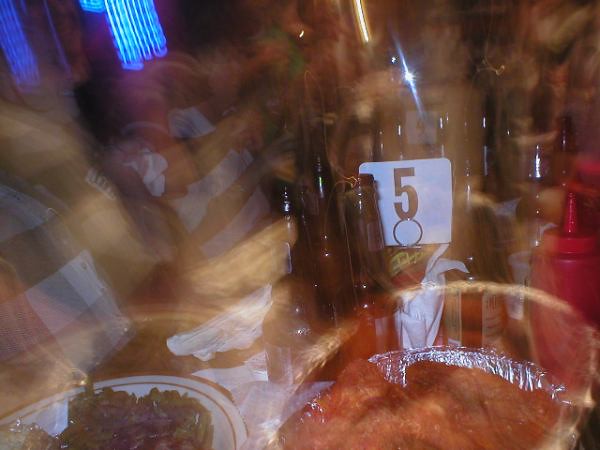This blurred and out-of-focus photograph, seemingly taken indoors, captures a scene at a restaurant or gathering. The image is distorted, possibly due to a glass pane in front of the camera. On the table, there are a few dark-colored beer bottles with long necks. A white square tag displaying the number five is visible near these bottles. Adjacent to the beer is a red squeeze tube of ketchup with a pointy top. In the foreground, there's a white plate with some dark, indeterminate food, positioned next to an aluminum foil container filled with reddish food. The upper left corner of the image faintly shows the bottom of a neon sign and some muted colors, including beiges, greens, and blues, which blend into the background. The scene includes people who appear to be looking upward, contributing to the impression of a busy, celebratory atmosphere.